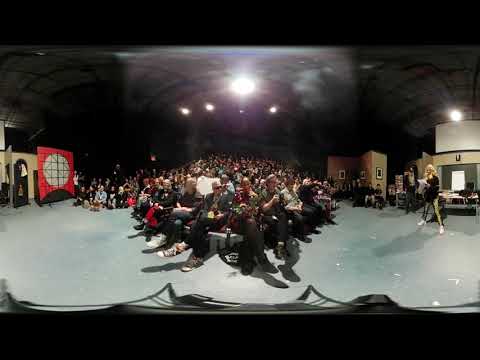This photograph captures a vibrant scene inside a large auditorium, distorted by a fisheye lens filter that curves the image and adds black horizontal strips to the top and bottom. At the center of the scene, a person holding a microphone appears to be either singing or giving a speech, engaging an attentive audience seated throughout the room, with a dense concentration in the middle. The auditorium features a grey floor and a dark, black designer ceiling, from which white lights shine down, illuminating the space. 

To the left, a door and a large red banner with white and intricate designs are visible, with a lady standing beside it. On the right, another lady stands with her legs apart, donning a black jacket and holding both a paper and a microphone, seemingly addressing the audience. Behind her, a man is present, and in the background, elements resembling office furniture or set designs suggest that this could be a studio audience on a movie or show set. The glare from the bright lights above adds a slight obscurity to the finer details, but the overall scene is lively and bustling with engaged spectators enjoying the performance or speech.